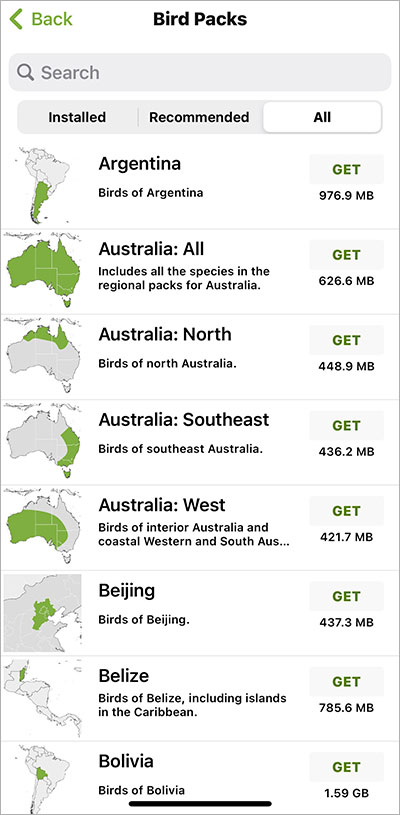The image displays a user interface for selecting bird packs from various regions. At the top, there is a green arrow labeled "Back". Below this, the title "Bird Packs" is prominently displayed. There's a search bar for finding specific packs, followed by tabs labeled "Installed," "Recommended," and "All," with the "All" tab currently active.

The interface lists several bird packs with detailed descriptions:

1. **Argentina**: Birds of Argentina - 796.9 megabytes
2. **Australia All**: Includes all species in the regional packs for Australia - 626.6 megabytes
3. **Australia North**: Birds of North Australia - 448.9 megabytes
4. **Australia South**: Birds of South Australia - 436.2 megabytes
5. **Australia West**: Birds of Interior Australia and Coastal Western and Southern South Australia - 421.7 megabytes
6. **Beijing**: Birds of Beijing - 437.3 megabytes
7. **Belize**: Birds of Belize, including islands in the Caribbean - 785.6 megabytes
8. **Bolivia**: Birds of Bolivia - 1.59 gigabytes

All text is in black font against a white background. Each entry includes a "Get" button in green. A map alongside each description highlights the specific region in green, set against a larger gray area for context.